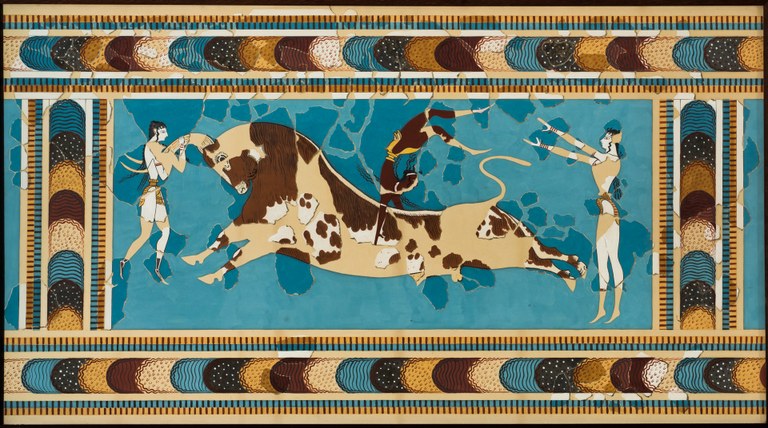This image showcases a detailed and vibrant reproduction of an ancient mural from the palace of Knossos in Crete. The artwork, set against a rich blue background framed with a tan border adorned with overlapping ovals in shades of blue, black, tan, brown, and cream, depicts a dramatic bull-leaping scene. At the mural's heart, a large, ornately painted bull in hues of tan, brown, and white dominates the image. In an impressive display of acrobatics, one figure is grasping the bull's long horns, another is caught mid-leap over the bull's back, and a third figure is positioned behind the bull, possibly in a motion to catch or toss the leaping acrobat. The scene is finely detailed, reflecting the ancient Greek artistic style, and illustrates a dynamic moment likely inspired by historical bullfighting events.